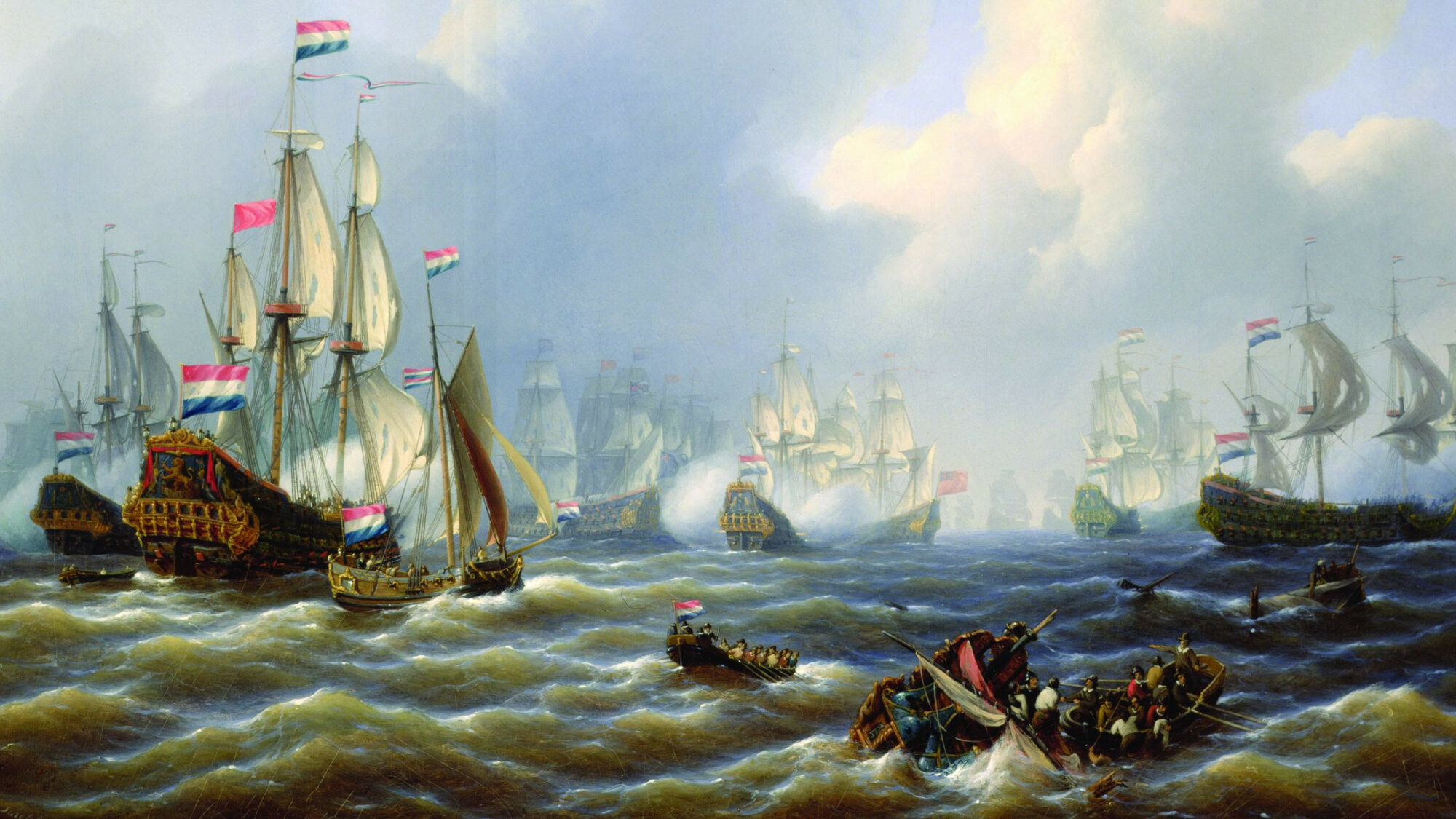This painting captures a tumultuous naval scene from what appears to be the 1700s, depicting a fleet of old wooden ships with large white sails battling on a choppy sea. The backdrop features a dramatic sky filled with white and grey clouds against a blue canvas, adding to the sense of chaos and movement. The ships, resembling frigates, are adorned with flags bearing horizontal red, white, and blue stripes, similar to the French flag, and some display solid red flags. The sea is particularly wavy, suggesting rough waters. In the foreground, several boats or small lifeboats are visible, filled with sailors and possibly soldiers, reinforcing the impression that a naval battle or war is taking place. The ships span across the composition, with some fading into the distance, hinting at the vastness of the scene and the intensity of the maritime conflict.